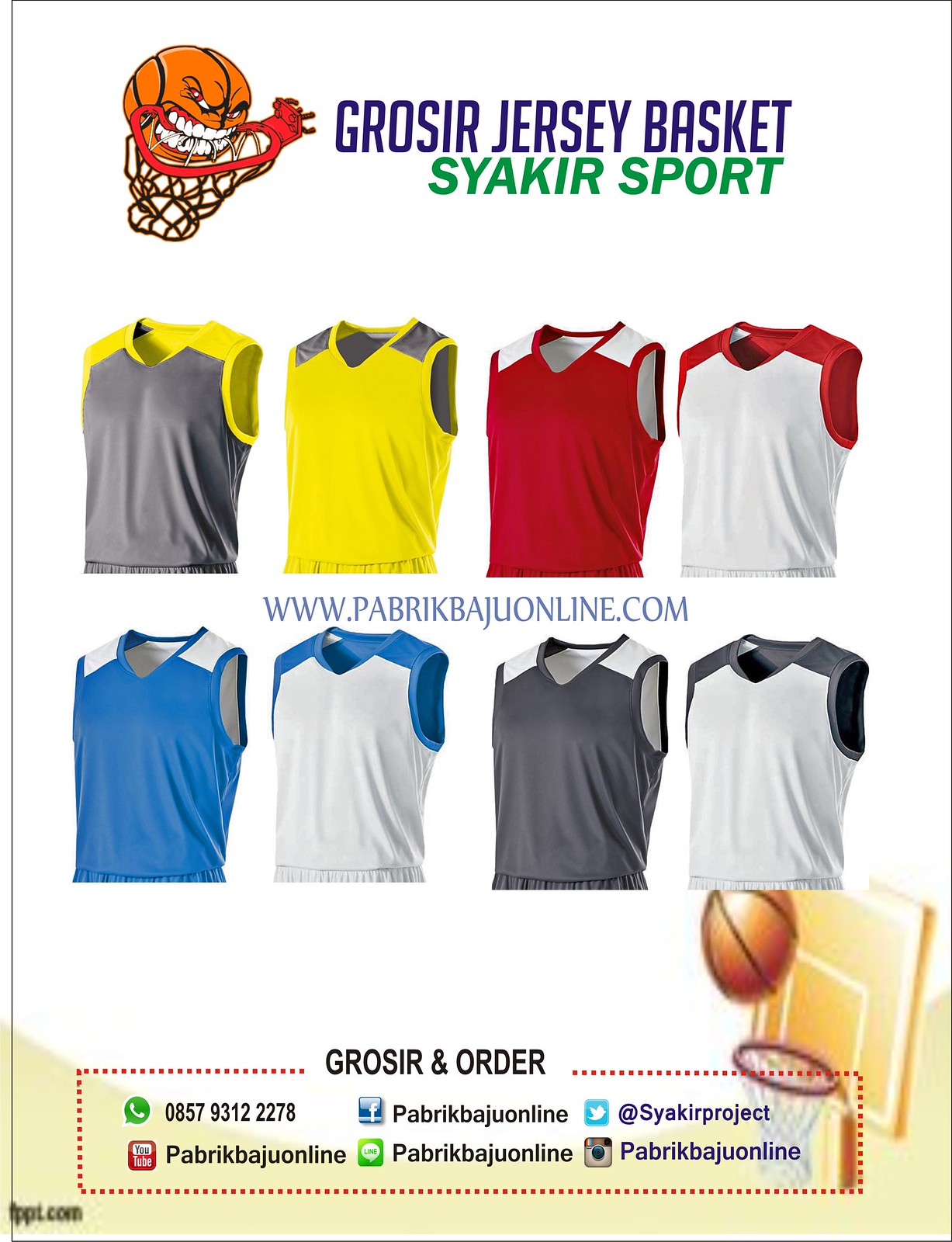This image features a promotional poster for an online sports apparel store with a vibrant red background. At the top left, there's a lively cartoon logo depicting a basketball with a face, complete with large white teeth, biting into the rim of a red basketball hoop, with a net hanging below the rim. To the right of the logo, in bold blue text, it says "Grocer Jersey Basket", and directly underneath in green text, it reads "Syakir Sport".

The poster prominently displays eight sleeveless athletic jerseys arranged in two rows of four. In the top row, the first jersey on the left has a gray chest with yellow shoulders, followed by one with a yellow chest and gray shoulders. Next is a jersey with a red chest and white shoulders, and lastly, a white chest with red shoulders. This pattern repeats in the bottom row but starts with a blue chest and white shoulders, followed by a white chest and blue shoulders. The next two jerseys in this row have a gray chest with white shoulders and a white chest with gray shoulders.

In the middle of the jerseys, the website "www.pabrikbajouonline.com" is displayed. Near the bottom, there's another image of a basketball with a hoop, and the border features a dotted red line. A section labeled "Grocer in order" contains contact details including a phone number and links to various social media platforms like Facebook (PabrikBajouOnline), Twitter (SyakirProject), Instagram, Line, and YouTube, signified by their respective logos.

This detailed poster effectively showcases the store's diverse range of vibrant athletic jerseys while providing all necessary contact information and web links to engage potential customers.